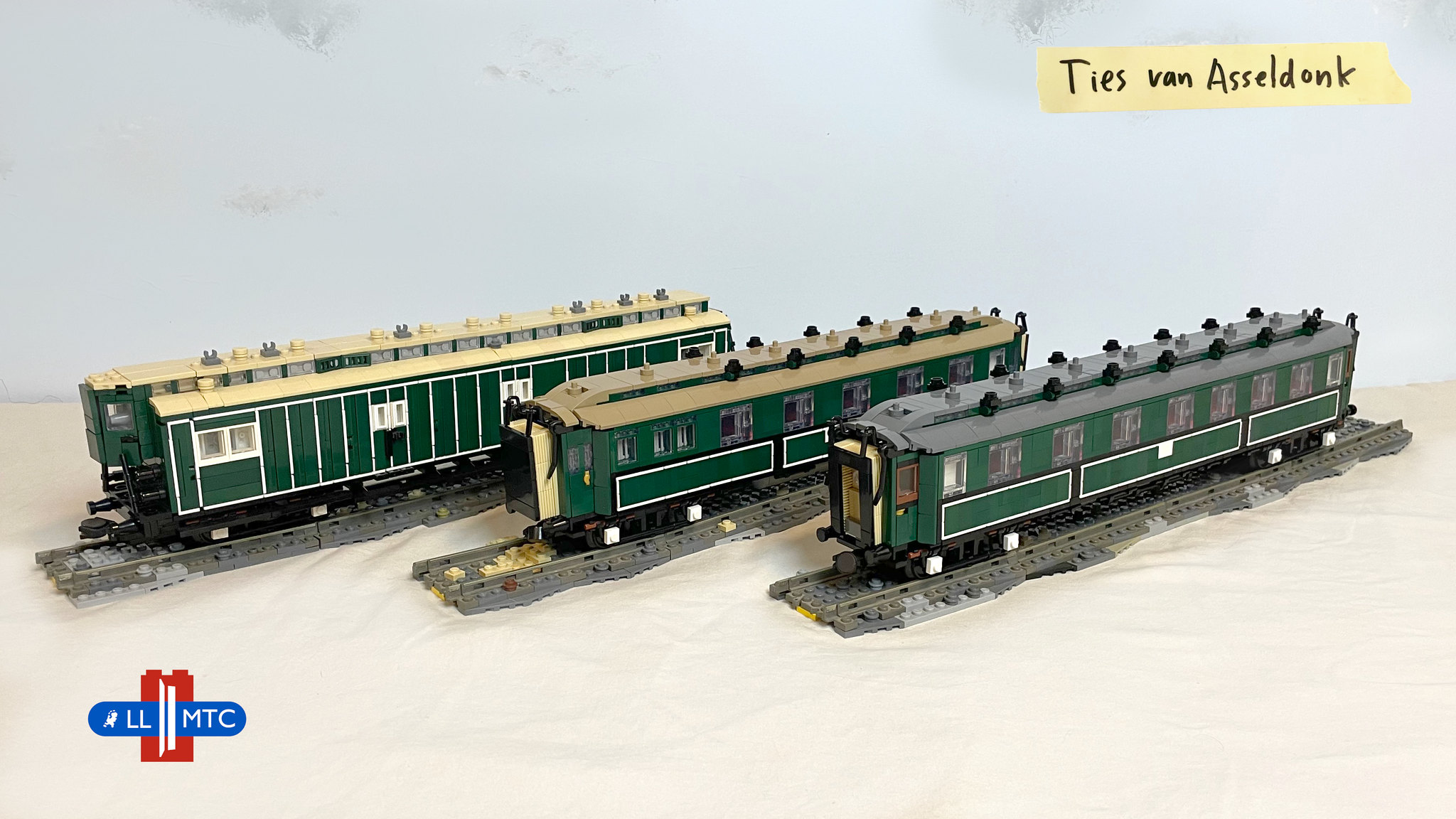The image showcases a detailed scene of three green model trains, each situated on its own individual track. The trains display varying roof colors: the leftmost train has a gray roof, the middle train sports a tannish beige roof, and the rightmost train features a pale yellow roof. They are all aligned at an angle to the left, allowing a clear view of both their fronts and sides. The tracks rest on a white, blanket-like surface. At the bottom left corner of the image, there's a company logo—a blue oval with the letters "LLMTC" in white, against a backdrop of a red brick tower. Near the top right, a yellow rectangle with the text “Ties van Asseldonk” is visible, resembling tape. The wall behind the trains appears white with some gray markings, completing the setting.